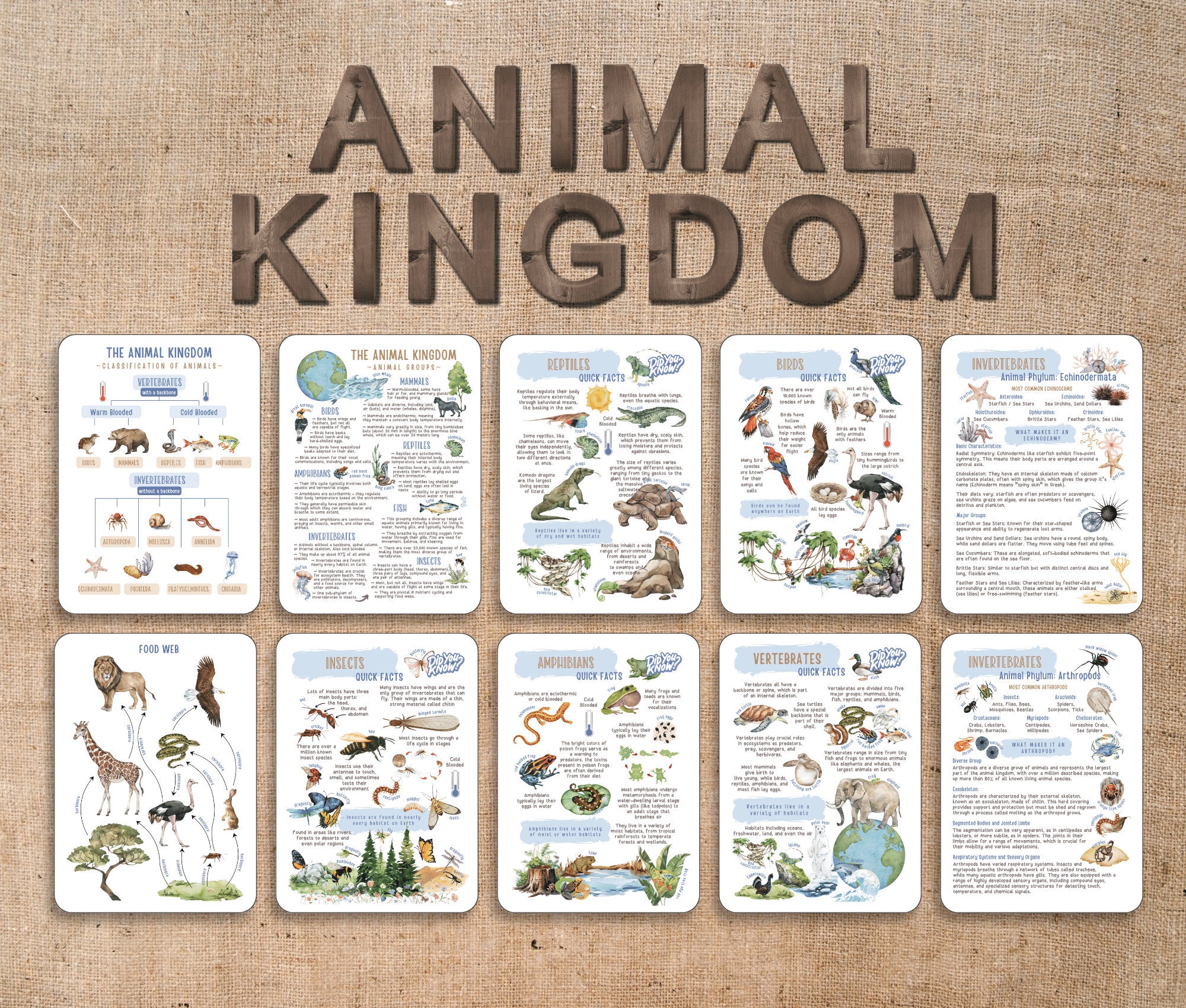The image displays a wall hanging or poster set on a textured background, possibly burlap or cork. Titled "Animal Kingdom" in a prominent brown heading, the display comprises ten letter-sized infographics, each on a white background and brimming with detailed information and colorful drawings about various animal groups. The first card classifies animals into categories such as vertebrates, invertebrates, warm-blooded, and cold-blooded species. The second card presents animal groups with illustrations of Earth, a tree, and various animals, further detailing mammals, birds, reptiles, amphibians, fish, invertebrates, and insects. Additional cards cover specific topics like reptiles, birds, amphibians, insects, and the food web, featuring quick facts, charts, and mini-drawings of animals such as dinosaurs, turtles, giraffes, sea turtles, alligators, and crocodiles. Each card provides rich textual information and visual aids, offering a comprehensive overview of the animal kingdom.